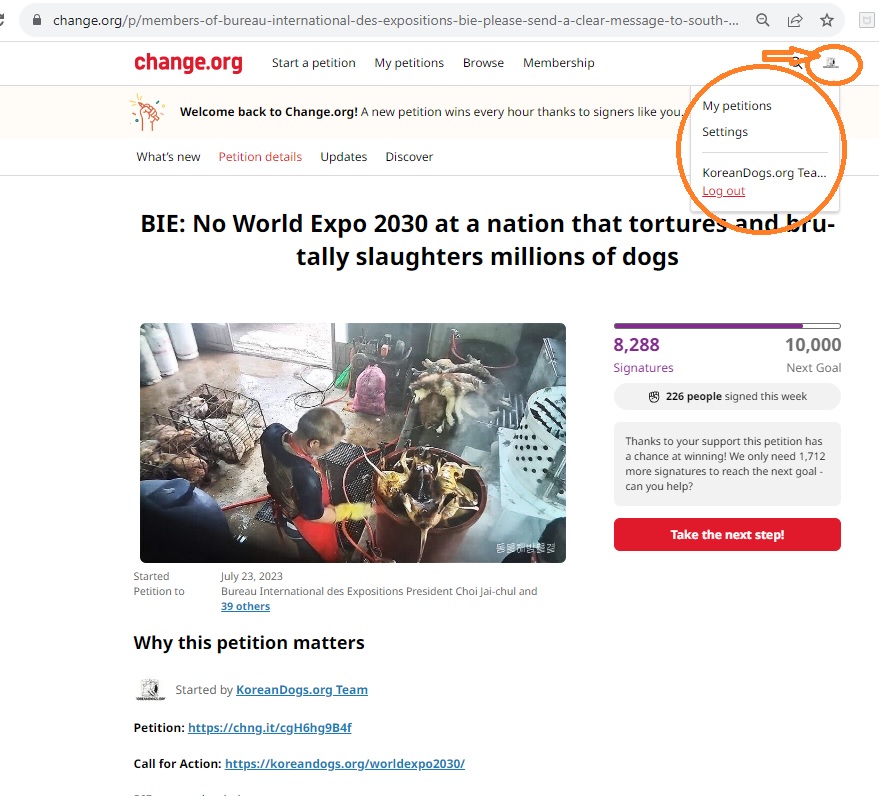The image displays a web browser interface featuring the website Change.org. At the top, the URL bar shows "change.org/p/members-of-bureau-international-des-expositions-PBIE-please-send-aid-clear-message-to-south...". Below this, the left-hand side of the screen prominently features the Change.org logo on a white background, accompanied by navigational tabs in black text: "Start a Petition," "My Petitions," and "Browse Membership."

A green arrow points to a small gray line with a black and white square box above it. A thin gray line stretches horizontally beneath this element. Further down, on a beige background, an orange hand holds a pencil beside bold black text stating, "Welcome back to Change.org!" Underneath, in regular black text, it reads, "A new petition wins every hour, day, so sign us like you." 

On the right-hand side, also on a white background, more black text reads, "In my petition sentence," followed by another thin gray line and "koreandogs.org, T-E-A,..." in black. The "Log out" option is highlighted in red and underlined, encircled by an orange hand-drawn circle. Below, in bold black text, there is an alarming message: "No World Expo 2030 at a nation that tortures and brutally slaughters millions of dogs."